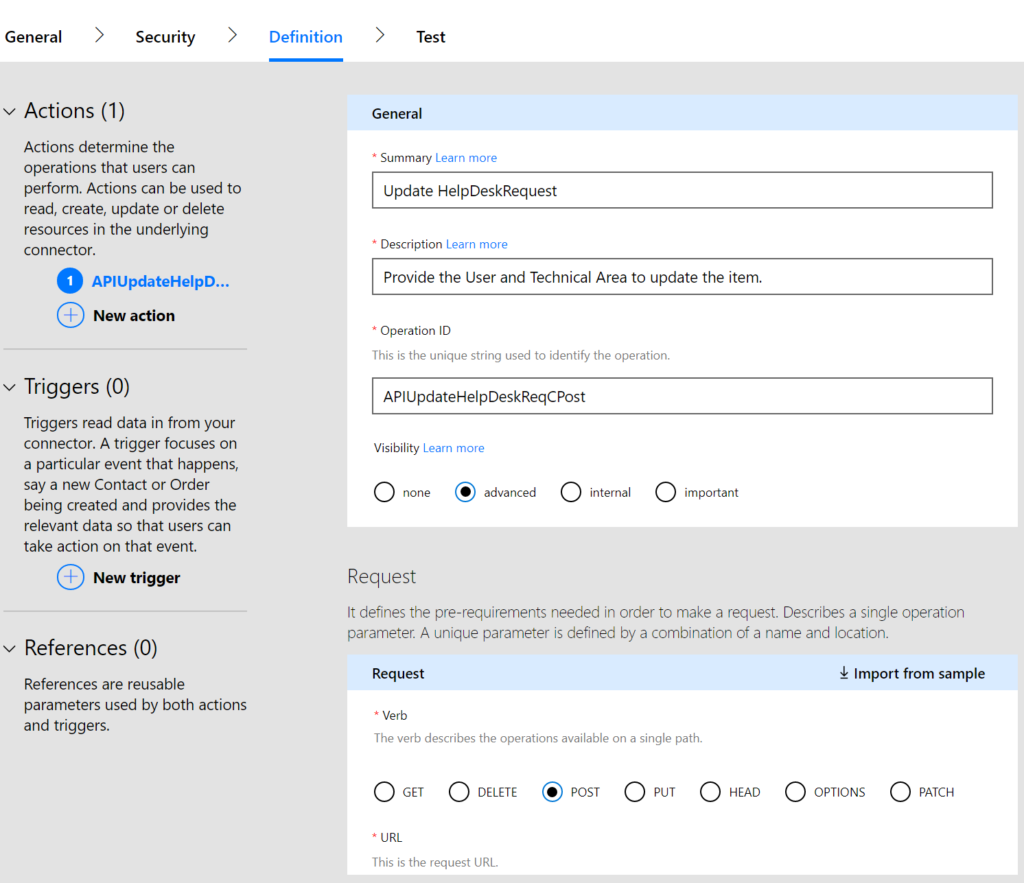A screenshot captures a web portal designed for configuring API options, showcasing fields for summary, description, operation ID, and HTTP request method. The left panel displays a guide on how to use the page, including sections for actions, triggers, and references. Meanwhile, the right panel features input fields and buttons for specifying API details.

In this instance, the user has already populated several fields: the summary is identified as "Update Help Desk Request," the description reads "Provide the user and technical area to update the item," and the operation ID is "APIHelpDeskRequestCPost." The user has set the API's visibility to "Advanced" and indicated that a POST request with a single parameter is needed. However, the request URL for the POST request has not yet been entered.

This step falls under the "Definition" phase of a multi-step process, which also includes steps for General, Security, and Test configurations. The background of the portal is predominantly gray, while the input boxes are placed within white divs, creating a clean and clear interface for users to complete their API setup.